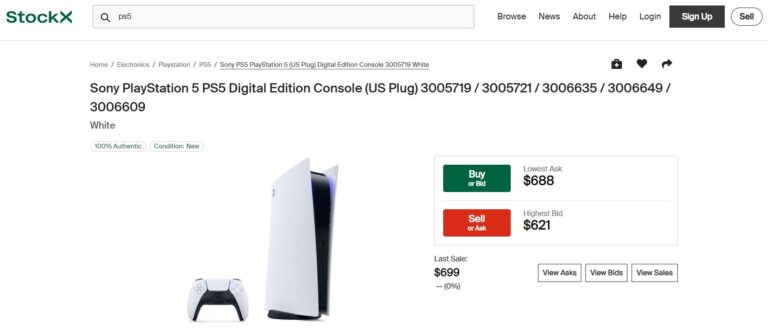This detailed screenshot from the StockX website captures the product page for the "Sony PlayStation 5 PS5 Digital Edition Console (US Plug)." In the top-left corner, the StockX logo features prominently in green letters. Centered at the top of the screen is a search bar with "PS5" entered. To the right of the search bar, a horizontal menu reads: "Browse", "News", "About", "Help", and "Login." Further right, a black "Sign Up" button with white text is positioned next to a circular white button with a black outline that says "Sell."

The main section of the screen is dedicated to the product details. The title at the top reads "Sony PlayStation 5 PS5 Digital Edition Console (US Plug)" with "White" noted just below in smaller text. A photo showcasing a white controller on the left and the PS5 console on the right is prominently displayed. To the right of the image, two stacked buttons offer purchase and sell options. The top green button reads "Buy or Bid – Lowest Ask: $688," while the red button below it states "Sell – Highest Bid: $621."